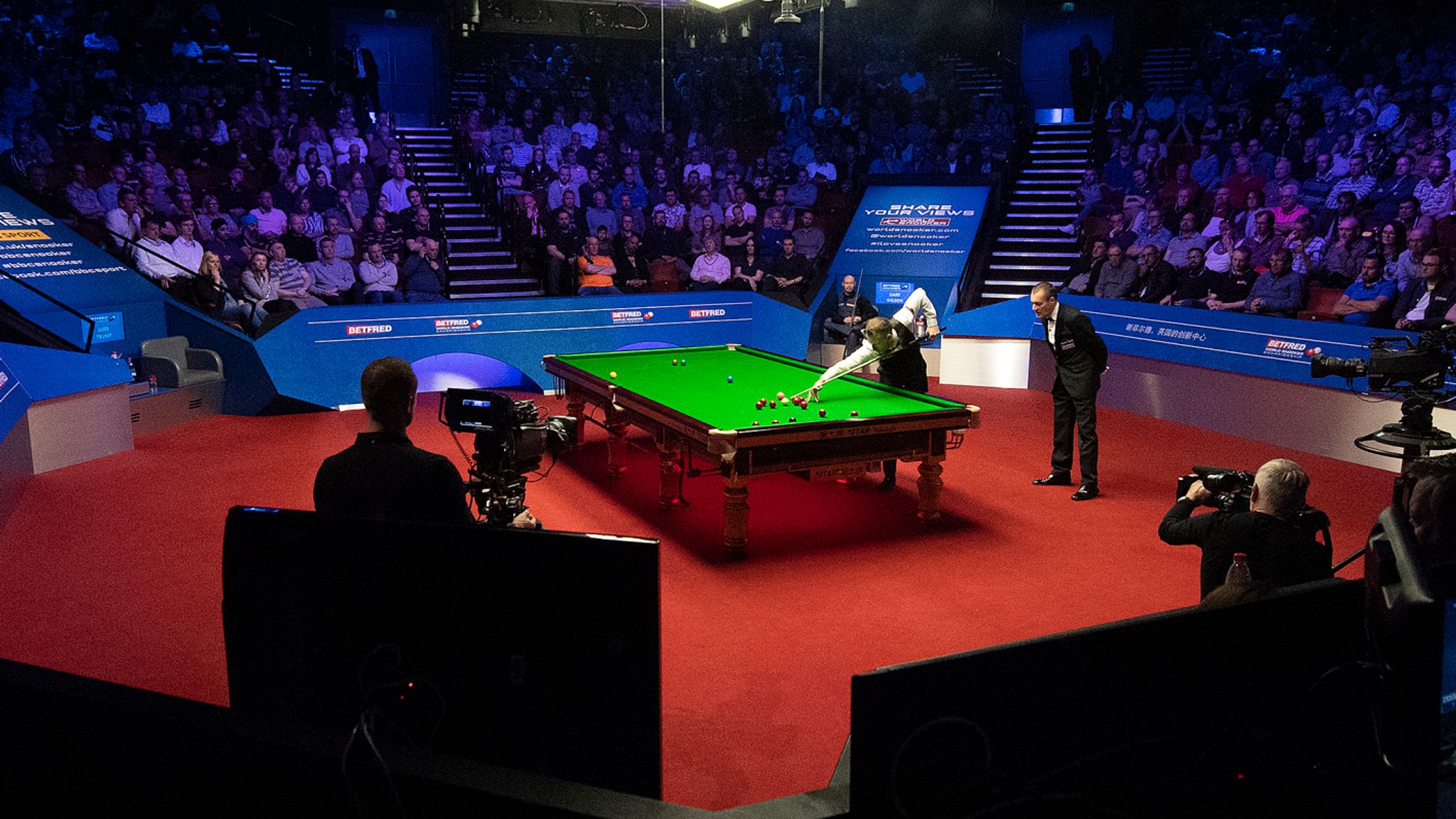The image captures a detailed scene of a televised pool tournament unfolding in a well-lit, studio-like arena. Central to the photo is a green-covered billiards table with a red carpet base, surrounded by blue banisters and scoreboards, making a vibrant contrast with the lighting focused on the table. A man in a white dress shirt and a tuxedo vest, with bands around his upper arms to keep the sleeves up, is poised to take a shot, evidencing the meticulous nature of the event. He appears to be playing left-handed, concentrating intensely on the cue ball. Nearby, a judge in a formal suit leans over, observing the shot closely. The opposing player, also dressed in formal attire, watches attentively from a seat behind the shooter.

The arena has a small, intimate feel with a full gallery of spectators in bleacher-style seating, accessible by stairways on either side. Multiple television cameras are positioned around the table, capturing every moment for the broadcast. The overall color scheme of the scene features reds, blues, green, and browns, complemented by the dimmed lights of the studio audience and the spotlights on the pool table. A sign in the background reads, "Share Your Views," indicating the interactive nature of the event. This combination of elements underscores the serious, competitive atmosphere of the tournament.